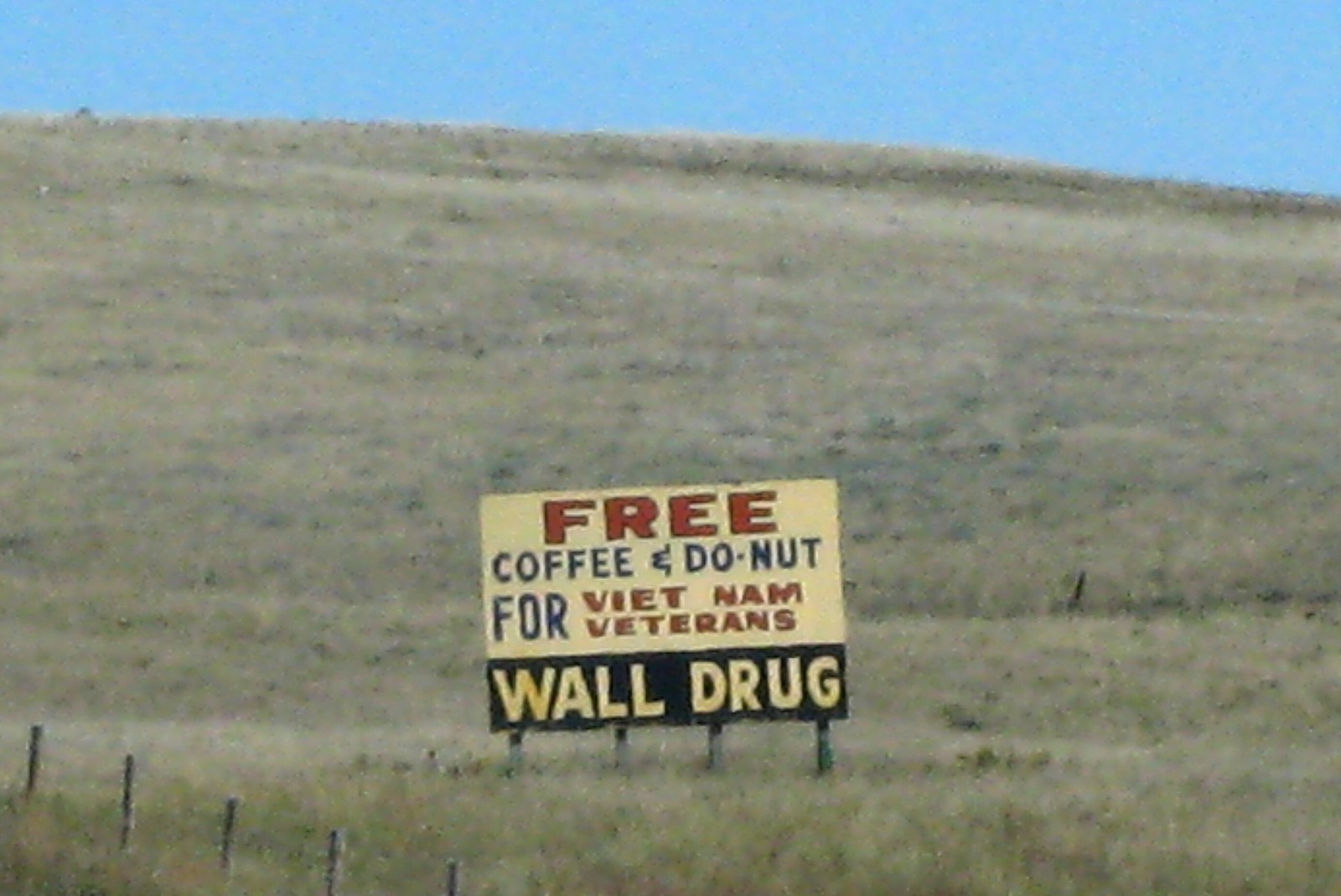In this grainy daytime photograph, an outdoor scene unfolds, capturing a hill bathed in the warmth of a pleasant climate. The hillside is covered in grass that displays a mix of green and yellow hues. In the lower left corner of the image, a fence made of wooden posts and strung with what appears to be barbed wire extends across the frame, though the details remain somewhat indistinct due to the image's graininess. Dominating the center of the scene is a vintage-looking sign, vividly colored in yellow and black with red and black print. It bears a message in block letters: "FREE COFFEE AND DONUT FOR VIETNAM VETERANS." Below this, set against a black background with yellow print, the sign reads "WALL DRUG" in capital letters. This retro sign is supported by four wooden posts, standing tall on the grassy hill. In the background, the horizon line is marked by a clear blue sky, completing the rustic and nostalgic ambiance of the photograph.